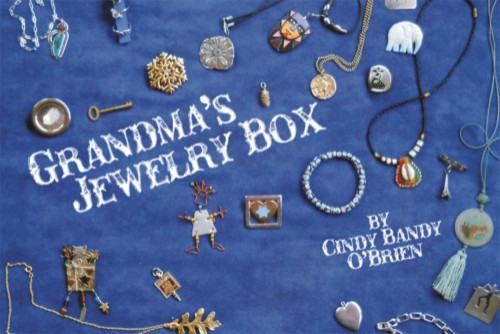This is a horizontally aligned rectangular image resembling a screenshot from a TV show or YouTube channel. The background is a dark ocean blue, textured like fabric. In bold, slightly faded white letters diagonally centered to the left, the title "GRANDMA'S JEWELRY BOX" is prominently displayed, with "Grandma's" above "Jewelry Box." In smaller white letters in the lower right corner, it says "by Cindy Bandy O'Brien."

The image is sprinkled with a variety of jewelry pieces and charms. Near the top, there is an old-fashioned gold brass key. A snowflake brooch, a turquoise necklace, a silver button, and a bracelet can also be spotted. Centered under the title lies an intriguing pin with an outline of a person, featuring a beaded head, a white trapezoidal body, and small beads for the arms and legs. A square pendant with a heart and a star inside it, and a beaded bracelet are placed thoughtfully.

Chains cascade from the upper right and bottom left corners. Some chains are beaded, while others are rope, each adorned with pendants, including a leaf pendant attached to a gold small link chain. Other items include a seashell necklace, an elephant pin, a heart-shaped charm, and an arrangement of additional pins scattered throughout. The details suggest a sentimental collection, artfully arranged to evoke nostalgia and curiosity.